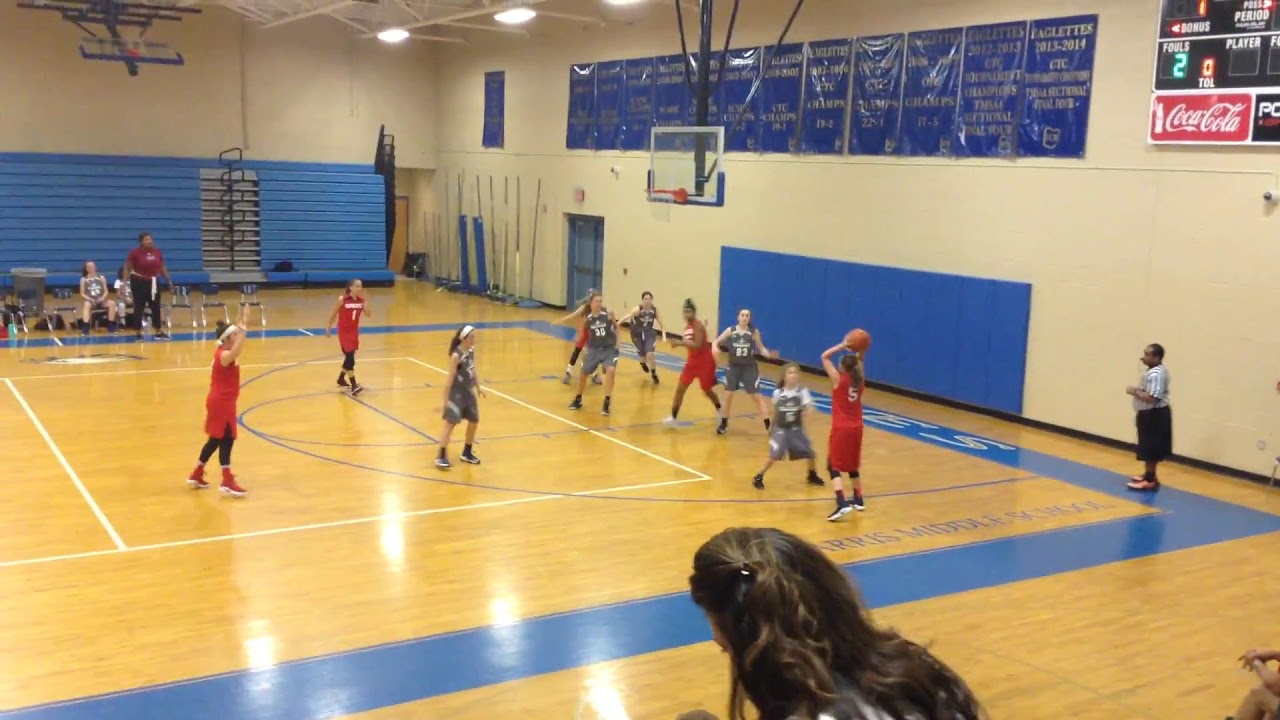The photograph captures a high-energy moment during a high school or possibly middle school girls' basketball game inside a gymnasium, with a clear vantage point from the stands. The court features a light parquet wood floor with blue and white outlines, suggesting team branding. The wall paint is a tan color, adorned with blue padding for safety. In the immediate foreground, the back of a brunette woman's head appears, hinting that the photographer is positioned in the spectator area.

On the court, the focal point is a player from the red team poised to take a shot from near the three-point line. Surrounding her are players from both teams, identifiable by their red and green jerseys. Interestingly, there's mention of both gray and blue jerseys, but the predominant colors seem to be red and green.

Positioned on the right side of the image, a referee, distinguishable in his black and white striped shirt and black shorts, stands attentively with a whistle in his mouth. He is a Black man, offering a visual contrast to the primarily white players, with one red team member who appears African-American.

In the background, there are partially pulled-out blue bleachers, with some spectators and a bench area where a couple of players from the green team are seated. A coach in a red shirt and black pants stands near the bench, actively engaged in the game. The scene is bathed in the characteristic lighting of indoor gymnasiums, capturing the intensity and excitement of the moment.